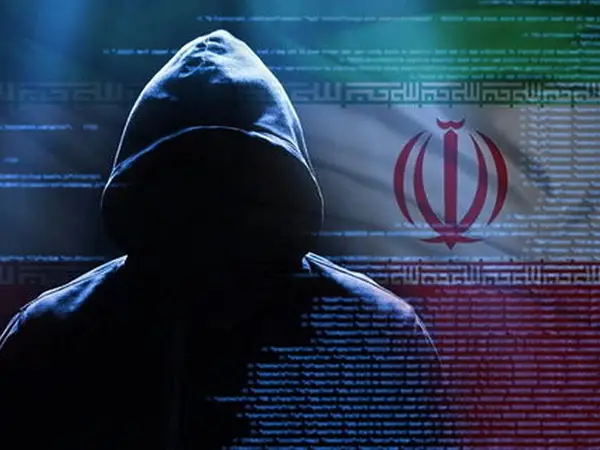The digital artwork presents an ominous and mysterious scene centered around a hooded figure with no visible face, shrouded in darkness where facial features should be. The person is cloaked in a dark grayish hoodie, which gently slopes down to chest level. The background features a striking and intricate design, resembling a foreign flag with horizontal stripes of green at the top, transitioning to teal and then gray in the middle, and finishing with a maroon or burgundy section at the bottom. Overlaying the flag are various symbols and writings in an unrecognized foreign language, adding to the enigmatic aura of the piece. The overall composition, with its blend of sinister and artistic elements, creates a powerful, haunting visual impact.